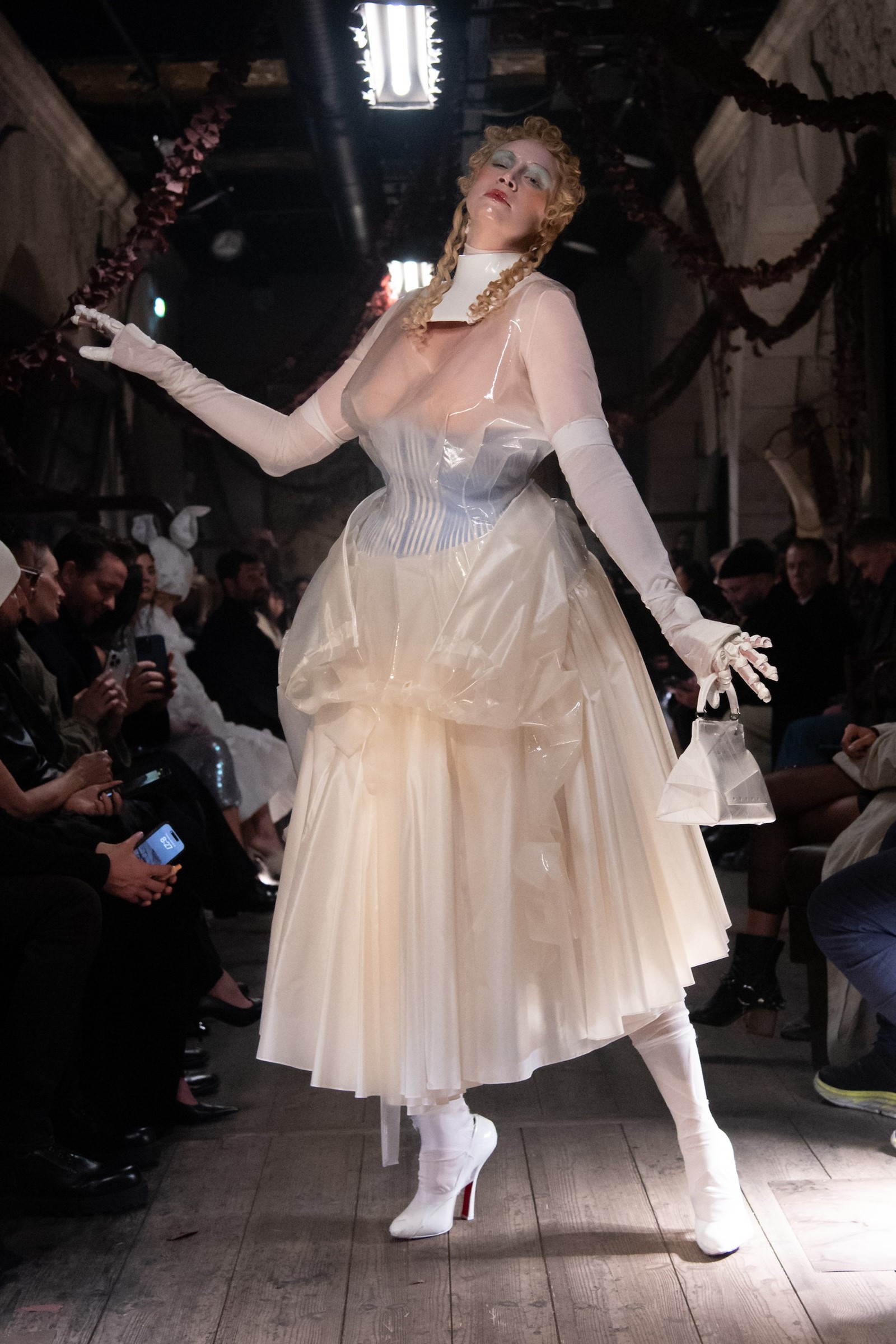The image shows a striking model, potentially a transvestite due to her imposing height and exaggerated features, standing on a wooden floor that serves as a non-traditional runway at a fashion show. Centrally positioned in the frame, she exudes elegance with her distinctive attire and pose. Her blonde, curly hair is styled into braided pigtails draped over her shoulders. She wears a Victorian-inspired outfit with modern twists: a sheer, white, possibly plastic dress that poofs out from just below the chest, revealing a blue and white bodice underneath. Her attire includes long white gloves extending to her biceps, high white socks, and white high-heeled shoes, with her right foot pointed on her toe and the left slightly out to the side. The model holds a small white bag in her left hand while her right arm extends gracefully. An illumination on the roof and wooden beams add depth to the scene, while rows of spectators, some with cameras or phones, fade into the distance on both sides, documenting the captivating display.